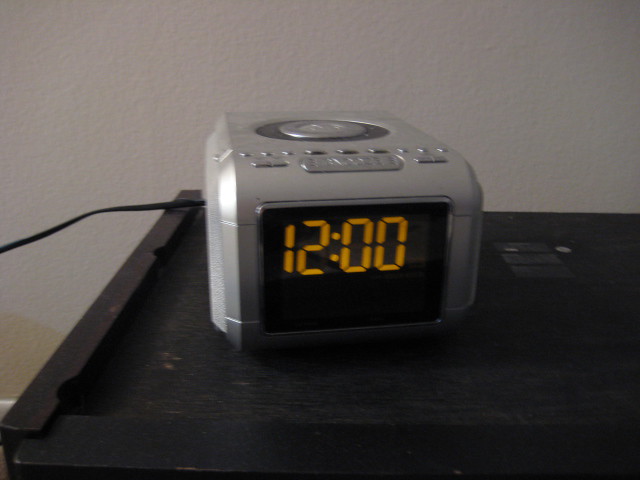This somewhat blurry image captures a vintage clock radio resting on a dark brown wooden side table. The clock radio has a silver body with a black face, featuring bright orange digital numbers that display the time as 12:00 PM. The top of the device appears to be equipped with a CD player, indicating that it may be an older model. Along the front of the clock radio, several buttons are visible, likely for adjusting the clock settings and tuning the radio. A power cord extends from the back of the radio towards the left, though the plug is not visible. The background features a plain, painted white wall, and there are no people or text in the photo.